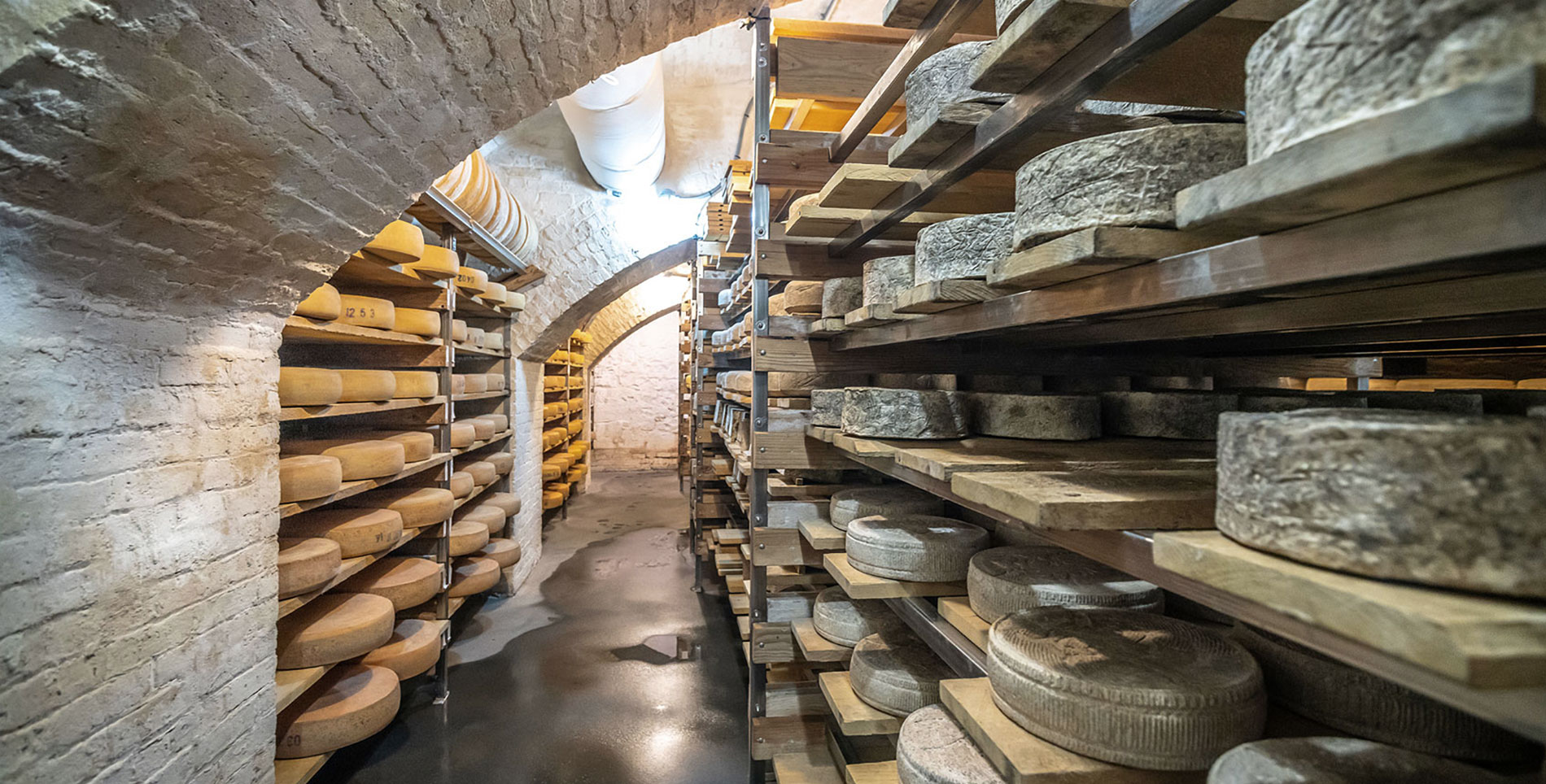This photographic image captures the view inside an indoor storage room, possibly a cellar or basement. The setting features a wet, gray cement floor with various puddles scattered along a central hallway. The hallway is flanked on both sides by metal shelves with wooden planks. On the right side, the shelves host numerous oval-shaped tins, possibly containing cheeses, with a variety of colors ranging from greenish moldy cheese on the top planks to blackish-gray cheese on the lower ones. 

The left side mirrors this shelving arrangement but with brown-colored items resembling wooden stumps or older cheeses, likely arranged on wooden slates. The atmosphere of the room suggests age and meticulous storage.

The room itself appears to be constructed from white bricks, evident in the curved walls and ceiling that give the space an arched appearance. Large, white-painted pipes run along the ceiling, contributing to the underground, industrial vibe of the setting. The arched brick walls and ceiling continue into the background, culminating in a white-painted wall, possibly with a doorway at the very end, reinforcing the enclosed nature of the space. Overhead, bright white lights illuminate the room, enhancing the visibility of the stored items. The overall ambiance is one of orderly storage, with a distinct juxtaposition of wetness and careful preservation of the contents on the shelves.